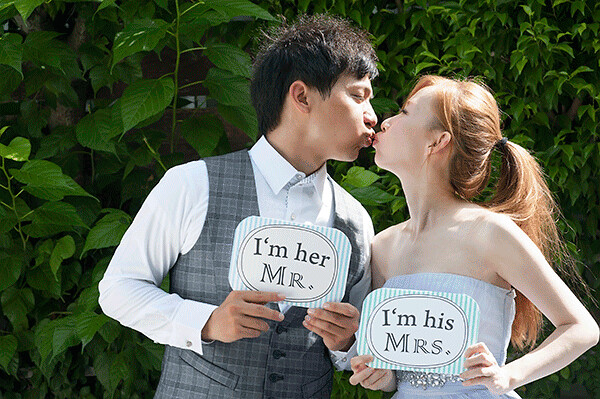In this full-color outdoor photograph taken on a sunny day, a young Caucasian redhead woman and a young Asian man share a kiss amidst a lush backdrop of green leaves. The image is wide and rectangular, capturing the couple standing in front of a thick layer of leafy plants, with larger teardrop-shaped leaves on the left and smaller, almost triangular leaves on the right. Behind the foliage, hints of a horizontal dark wooden fence are visible, adding depth to the scene.

The couple is positioned in the center, with their bodies facing forward but their heads turned towards each other for the kiss, showing the sides of their faces. The man, with short brown hair, sports a white button-up shirt beneath a gray plaid vest. He holds a speech bubble sign with vertical blue and white stripes, reading, "I'm her Mr." The woman, with her reddish hair pulled back in a ponytail secured by a black ponytail holder, wears a light blue sleeveless dress that may have a rhinestone detail at the waist. She holds a matching sign that says, "I'm his Mrs." The scene suggests they are celebrating a significant event, such as a wedding or an anniversary, adding to the charming and delightful nature of the photograph.